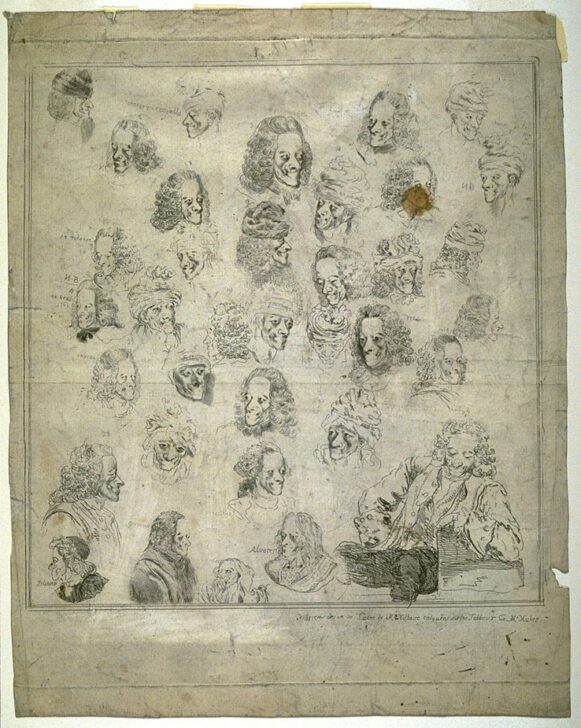This image appears to be a meticulously drawn collection of black and white pencil sketches on what looks like an old linen or parchment paper, possibly from the era of Benjamin Franklin. The paper, a vertical rectangle with a visible inner rectangle outline, features numerous detailed representations of a man from various angles, showcasing his distinctive curly hair with a thinning top, reminiscent of 18th-century hairstyles. The gentleman's portraits include forward-facing and side profiles, with some images showing him wearing different types of hats, including a turban. The bottom row of the sketches depicts more than just the head, revealing parts of the shoulders, with one figure donning a black suit and another in a half-body pose wearing a draped, old-fashioned attire. Faint black writing is present towards the lower right corner of the parchment, though it's too small to decipher. The paper appears to hang on a light gray surface, adding to its antique aura.